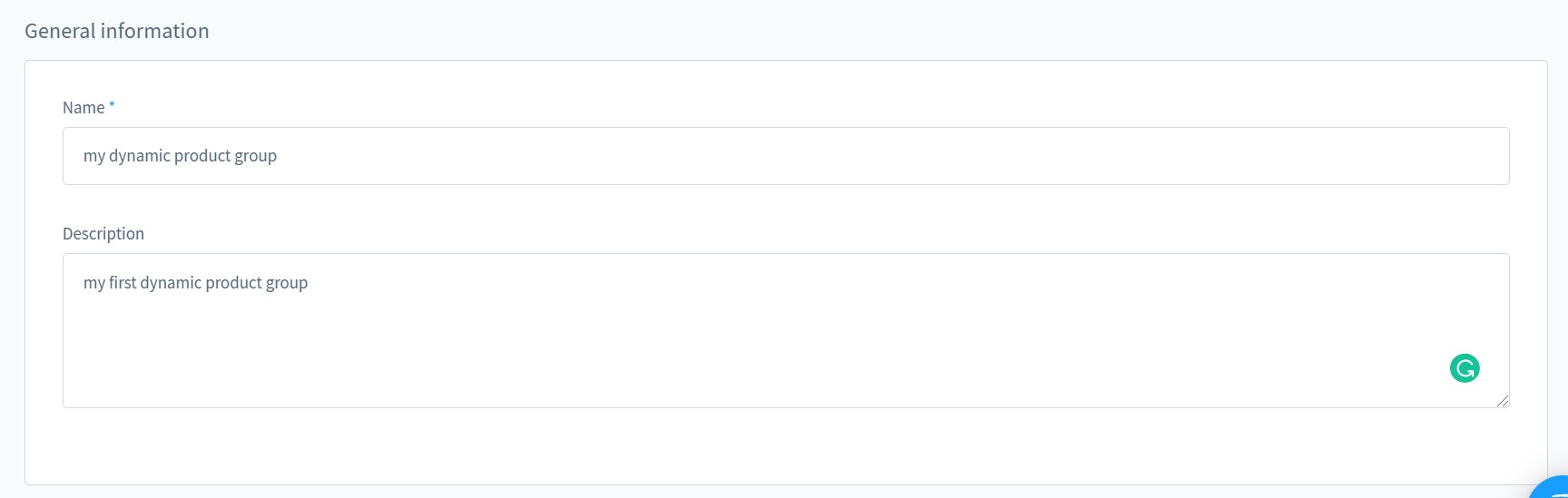The image has a four-to-one width-to-height ratio, with a light gray background. In the upper left corner, "General Information" is written in left-aligned black text, with the "G" in "General" capitalized.

Beneath this section, a prominent white box occupies the majority of the image. Inside this white box, starting at the top left, "Name" is displayed in black text with the "N" capitalized, followed by a small blue star in the upper right corner of the text.

Directly below "Name" is a lengthy text entry box, capable of accommodating long inputs. The text entered here reads "My Dynamic Product Group."

Further down, the word "Description" is written in left-aligned black text with the "D" capitalized. Below this label is a larger text box, approximately three times the height of the name entry box but equally as wide. In this box, the description "My First Dynamic Product Group" is typed.

In the bottom right corner of the description box, a medium green circle features a curved arrow, starting at the one or two o'clock position and looping around to the three-thirty position, symbolizing a refresh or update function.